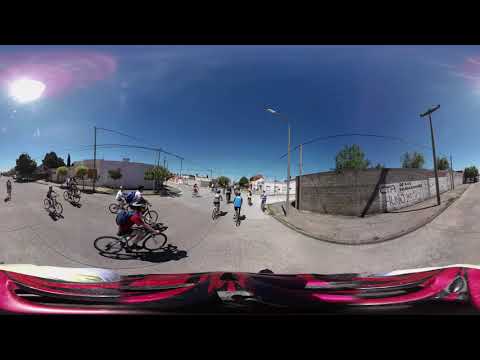This outdoor photograph, captured with a fisheye or wide-angle lens, presents a bustling street scene teeming with cyclists. The curved perspective of the image gives the impression of streets bending and merging into one another, typical of a panoramic shot. Numerous cyclists, donned in biking helmets, navigate the concrete road that runs the entire length of the photo, with one cyclist in a blue shirt riding away from the camera and another in a red t-shirt prominently positioned in the center. A rider with a white hat also draws attention. The roads and sidewalks, both a uniform gray, frame the scene, enhanced by additional details such as a graffiti-adorned single-story building and several telephone or power poles. On one side, a streetlight stands unlit against the vivid, darkish blue sky, while distant white signs punctuate the horizon. The sun, a bright white orb, rests high in the top left corner, casting a glow over a seemingly sparse, urban landscape.